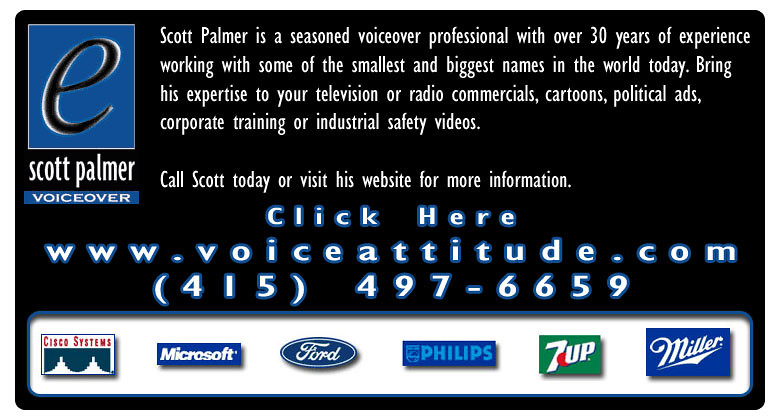The image appears to be an advertisement or business card for Scott Palmer, a seasoned voiceover professional with over 30 years of experience. The top portion features a black background with a blue section containing a black cursive lowercase 'E' on the far left. The text next to it introduces Scott Palmer and highlights his extensive experience working with both small and major companies worldwide. The text reads, "Scott Palmer is a seasoned voiceover professional with over 30 years of experience working with some of the smallest and biggest names in the world today. Bring his expertise to your television or radio commercials, cartoons, political ads, corporate training, or industrial safety videos."

Further details include a call to action: "Call Scott today or visit his website for more information," followed by clickable text, "Click here," with the website address www.voiceattitude.com and a phone number (415) 497-6659. The bottom of the image features a white rectangle with several corporate logos, likely representing companies Scott has worked with: Cisco Systems, Microsoft, Ford, Philips, 7-Up, and Miller. The overall design is set on a black background.